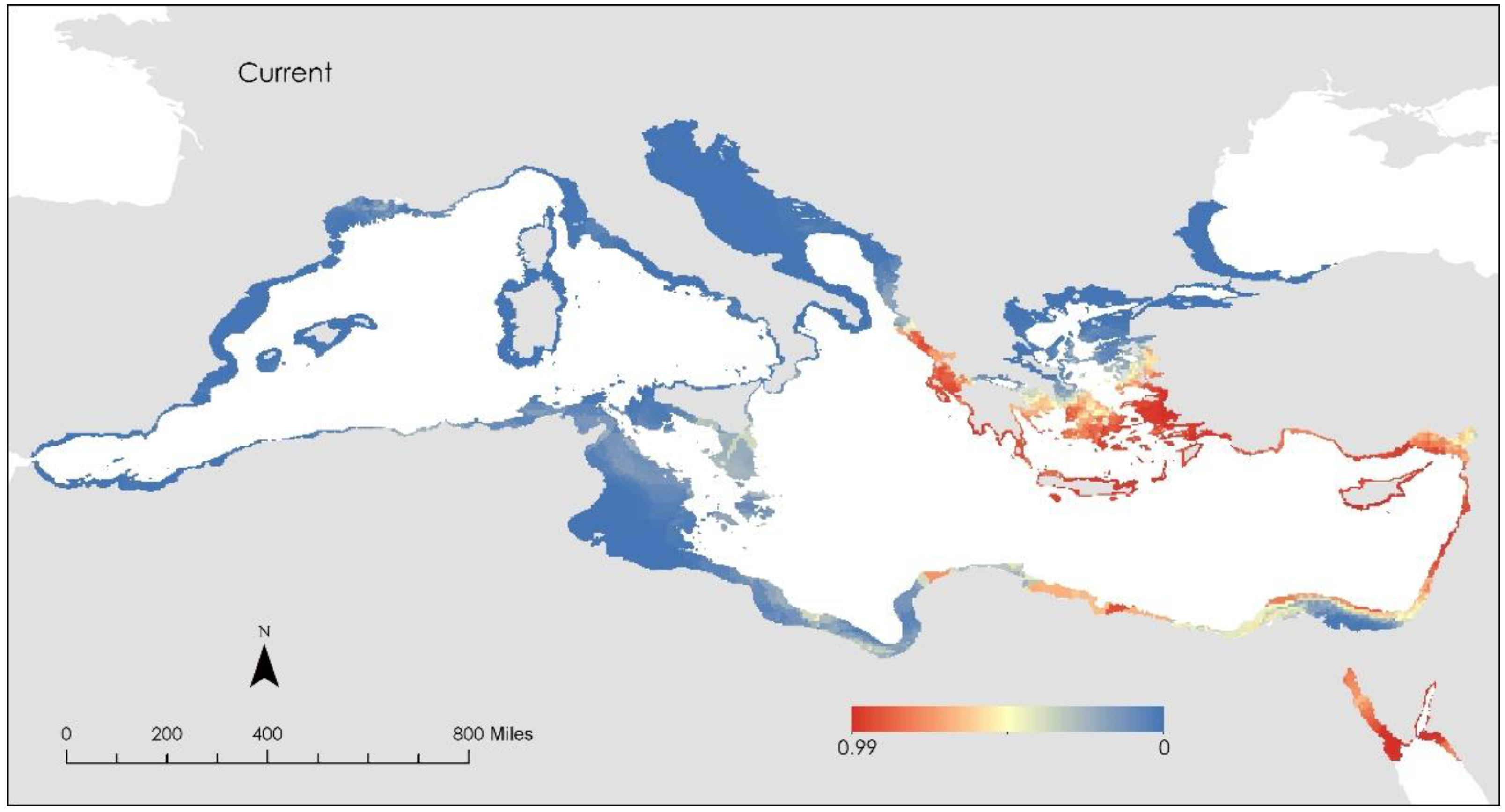This image depicts a scientific diagram, possibly a map, with indistinct white landmasses set against a gray background. The map prominently features two amorphous islands, each outlined with a gradient of colors ranging from dark blue to red. The borders of these landmasses transition through a spectrum from blue to red, indicating varying data points. In the top left corner, the word "current" is displayed. At the bottom, a color gradient chart ranges from zero (blue) to 0.99 (red), suggesting a scale of measurement. Additionally, a compass-like scale in the bottom left corner indicates distances from zero to 800 miles, with a northward pointing arrow. The map's intricate details, such as the colored borders and gradients, highlight particular data variations around the coastlines of these otherwise unidentifiable landmasses.